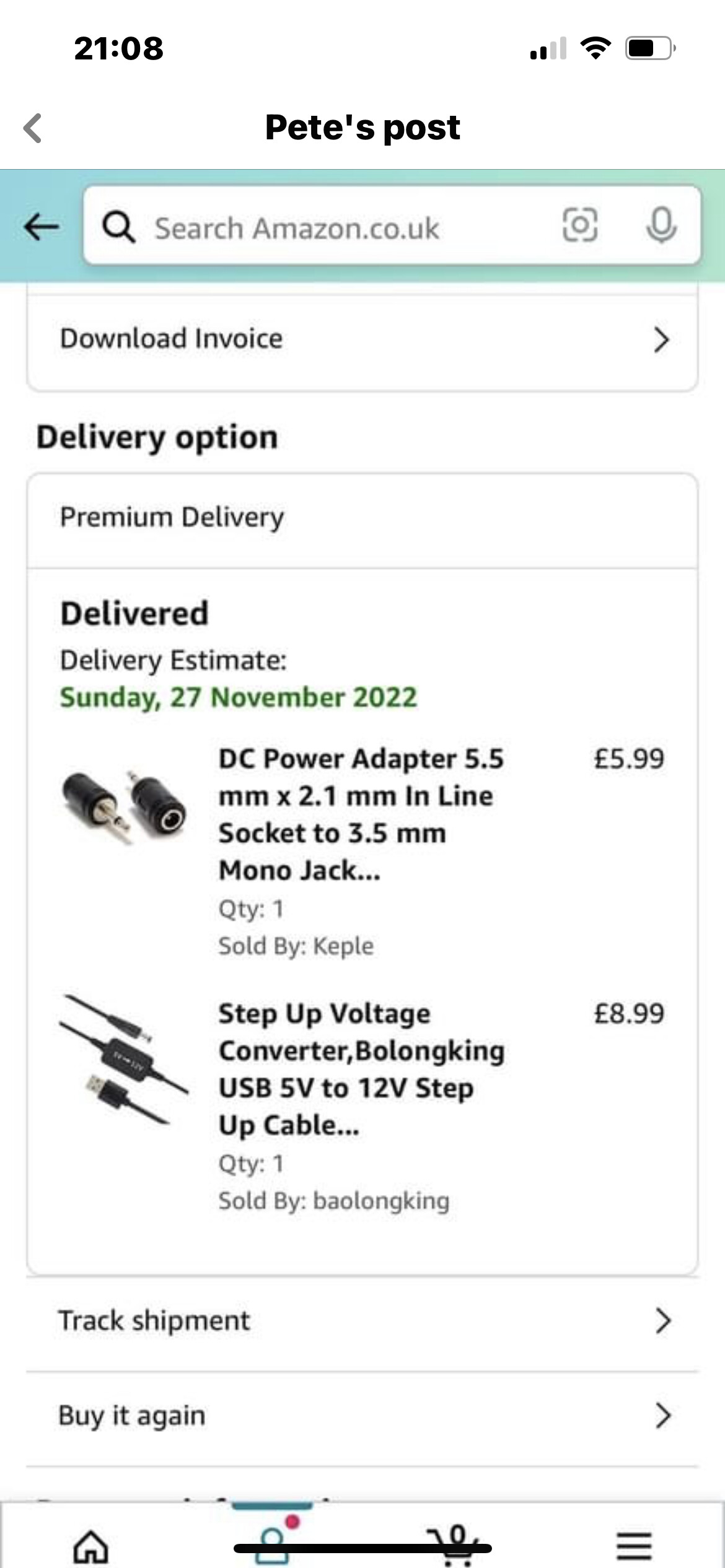This image is a screenshot of an Amazon UK page viewed on a mobile device. The page falls under the category "Pete's Post" as indicated at the top. Beneath this, there's the address bar showing the Amazon UK URL. The screenshot specifically displays the delivery options for two purchased items: a DC power adapter and a step-up voltage converter. The estimated delivery date for these items is Sunday, November 27th, 2022. The DC power adapter is priced at £5.99, while the step-up voltage converter costs £8.99. At the bottom of the page, there are options to track the shipment and repurchase the items.